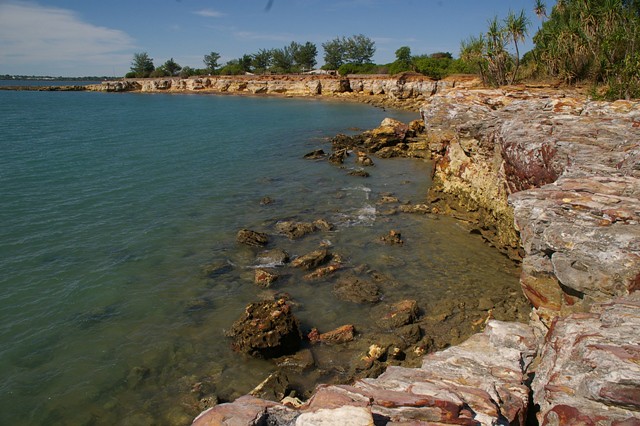The image captures a picturesque cove on the shores of a tropical body of water, possibly a large lake or an ocean bay. The shoreline is composed of an array of red, gray, and white rocks that form a natural barrier between the clear, blue-tinted water and the lush greenery. On the right side, thin, spindly green trees stand amidst towering palm trees, contributing to the tropical ambiance. Jagged rocks protrude from the water about 10 feet from the shore, enhancing the rugged beauty of the scene. The cove wraps around like a small bowl, curving gracefully around the translucent water. At the distant background of the image, atop a cliff adorned with additional palm trees, there is a small house. The sky is clear with very few clouds, allowing the vivid colors and details of the landscape to shine through. Additionally, a small jetty can be seen in the top left corner, extending modestly into the serene waters.